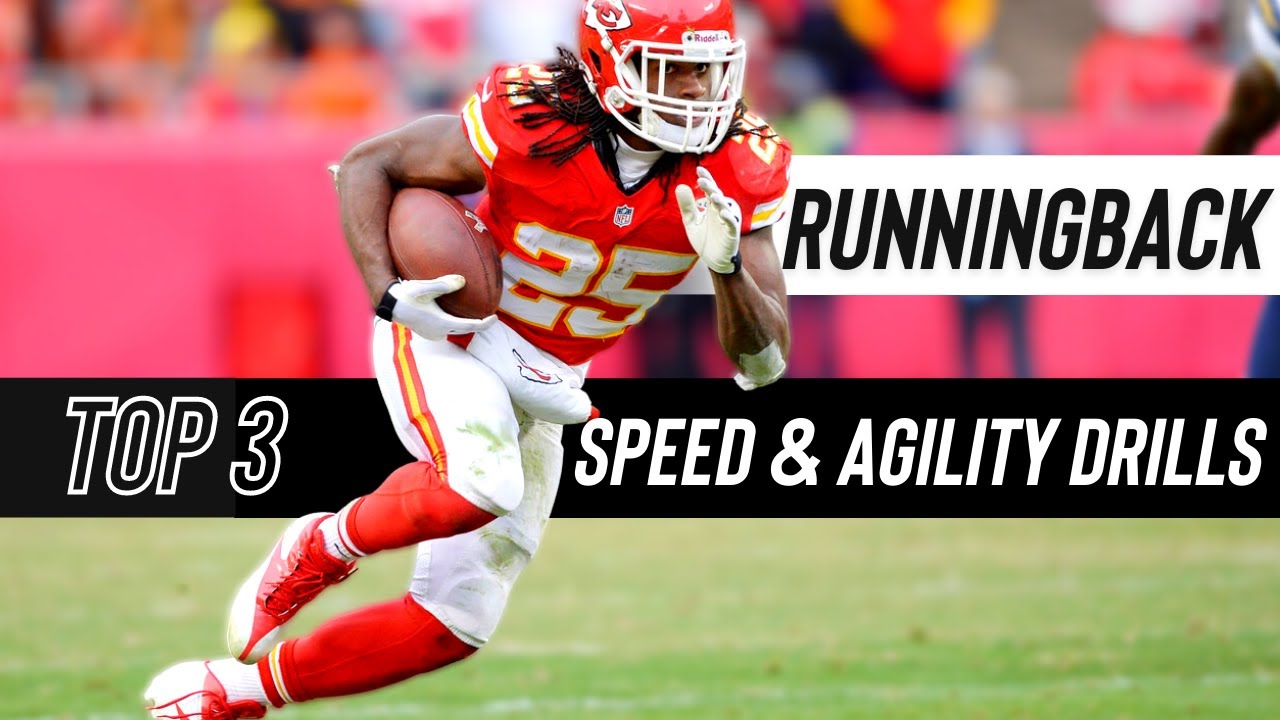The image captures a dynamic photograph of an African-American college-age football player in mid-sprint on a grassy field, presumably taken during a game. The player is wearing a complete Kansas City Chiefs uniform, which includes a bright red helmet with a white face mask, a red jersey featuring the number 25 with yellow and white stripes, and fully white pants accented with yellow and red stripes down the sides. His attire is complemented by red socks and red and white sneakers. He holds a football firmly in his right arm, while his left hand is bent and pointed up toward his chin. His long, braided hair can be seen spilling out from under his helmet.

The background of the image is blurred, highlighting the player against a mixture of green turf and a red backdrop, likely composed of the stadium's crowd and sidelining equipment. Overlaying the photograph are two text banners: a white banner with black letters reading "RUNNING BACK" appears on the right, and a black banner with white letters across the bottom states "TOP THREE SPEED AND AGILITY DRILLS."

The player is captured in a three-quarter view, with his left foot grounded and his right foot mid-motion, embodying speed and athleticism, suggesting that this image could be a cover for a video on YouTube showcasing the top three speed and agility drills for running backs.